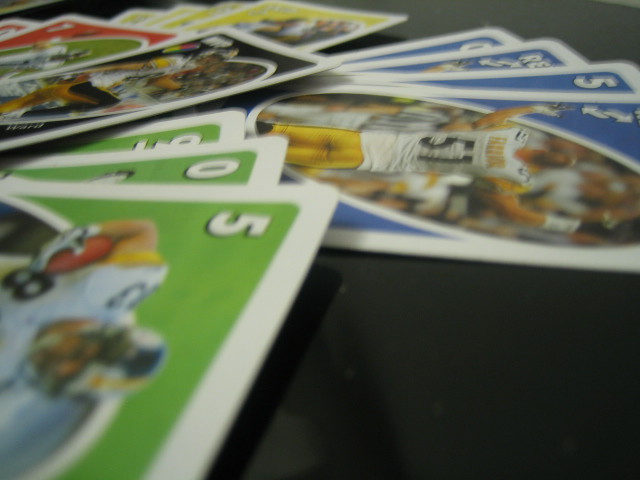In this image, there are several sets of sports-related cards prominently displayed on a black table. Each card features an American football player in various poses and is distinguished by different background colors and numbers in the top left corner. There are three green cards showing the numbers 5, 0, and 9. A set of four blue cards includes numbers 5 and 0, along with one card featuring the letters 'RE' and two arrows, one pointing up to the right and the other down to the left, possibly indicating the word "rest." Additionally, there are four yellow cards and one singular black card. The detailed arrangement and color differentiation suggest these cards are part of a collectible or gameplay system, each card representing distinct values and actions within the game.